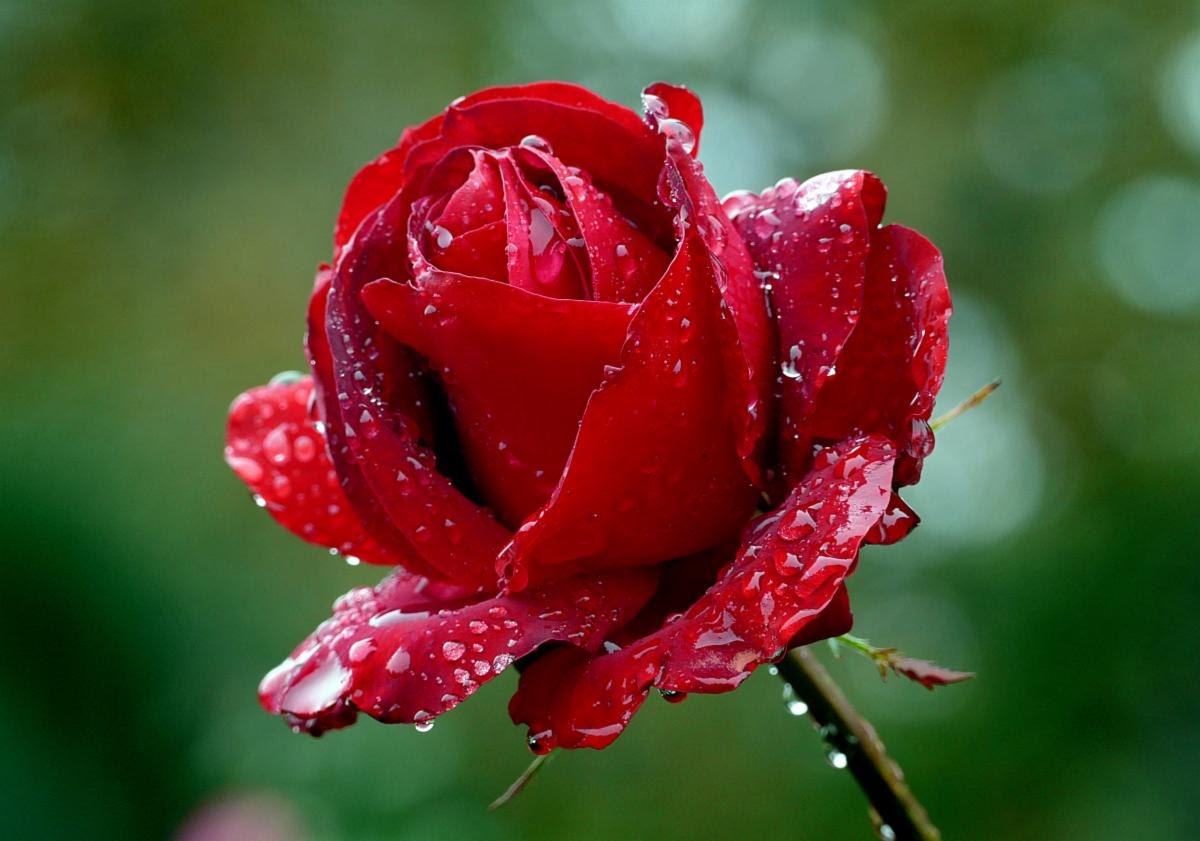This highly detailed, close-up image captures a vibrant red rose, its petals adorned with crystal-clear water droplets. The macro shot focuses on the rose’s rich, deep red petals, some of which fan out loosely around the central, tightly wrapped bud. Tiny green leaves peek from the bottom edge, and the green stem, also dotted with shimmering water droplets, extends downward. The background, a blurred expanse of dark green with soft, white bokeh circles, places full emphasis on the striking beauty of the rose. The entire composition exudes a sense of freshness, reminiscent of a recent rain, showcasing the rose in exquisite detail.